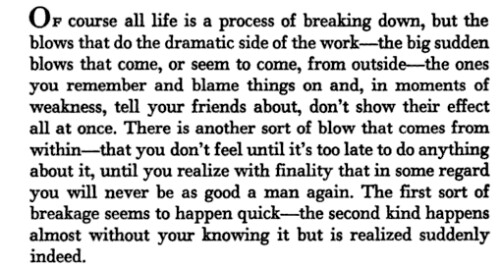The image features a densely written paragraph of text in black font against a plain white background. The paragraph, which appears to be excerpted from a book, delves into the theme of life and the process of breaking down. It portrays two types of blows that break a person down: the sudden, dramatic blows from external sources that are remembered and blamed for troubles, and the insidious, internal blows that go unnoticed until it's too late, marking a permanent change in one's character. The text describes how the first type of breakage seems to occur quickly and overtly, while the second type is gradual and subtle, only realized with a sudden, painful clarity. The paragraph underscores a profound life lesson about the nature of personal breakdowns and their inevitable, yet differing impacts.